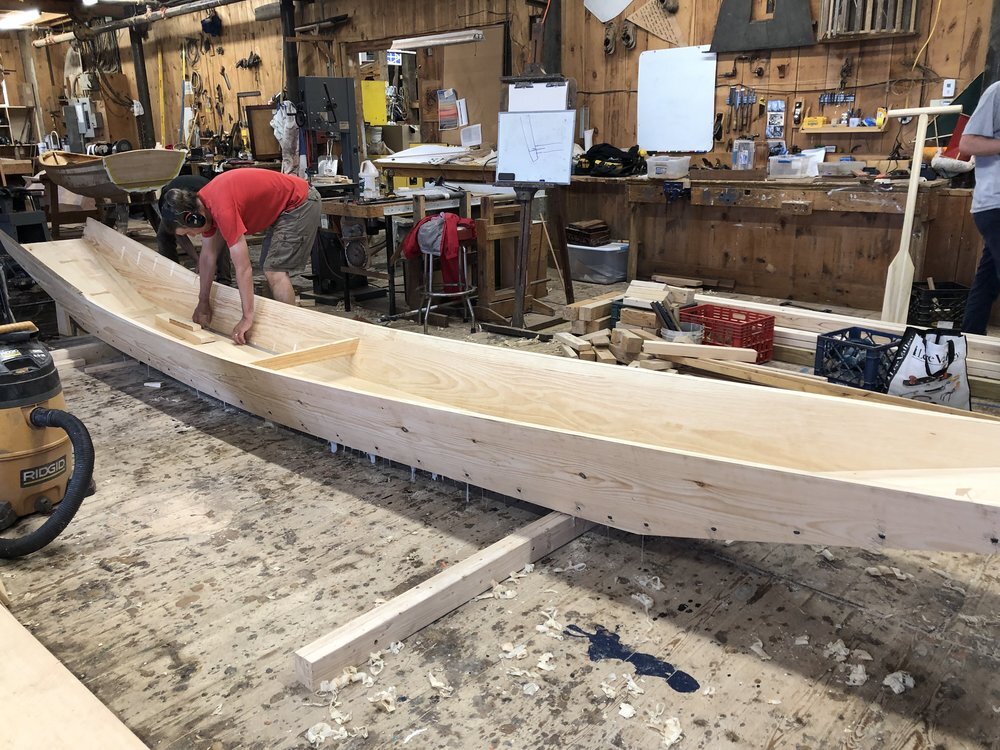In the bustling interior of a woodworking shop, a man in a red t-shirt and grayish cargo shorts is intensely focused on crafting a long and slender wooden rowboat, almost reminiscent of a kayak but capable of fitting several people. The boat remains in its raw, unstained wood form as the man methodically glues and secures the various pieces together, bent over to precisely align the edges and ensure structural integrity. Strewn across the floor around him are wood shavings and scraps, alongside a yellow shop vac with a black hose, positioned to his left.

The workshop is an organized chaos of tools and materials. Wooden-paneled walls and a sturdy workbench form the backdrop, where numerous tools hang in rows, and blueprints and white sheets on easels hint at ongoing designs and plans. Another partially visible person in a gray t-shirt can be seen walking away to the right side of the image, near wooden oars and more scattered tools. Further to the left, in the background, a more traditional-looking boat is noticeably elevated. The environment exudes a sense of dedicated craftsmanship and the meticulous nature of boat building.